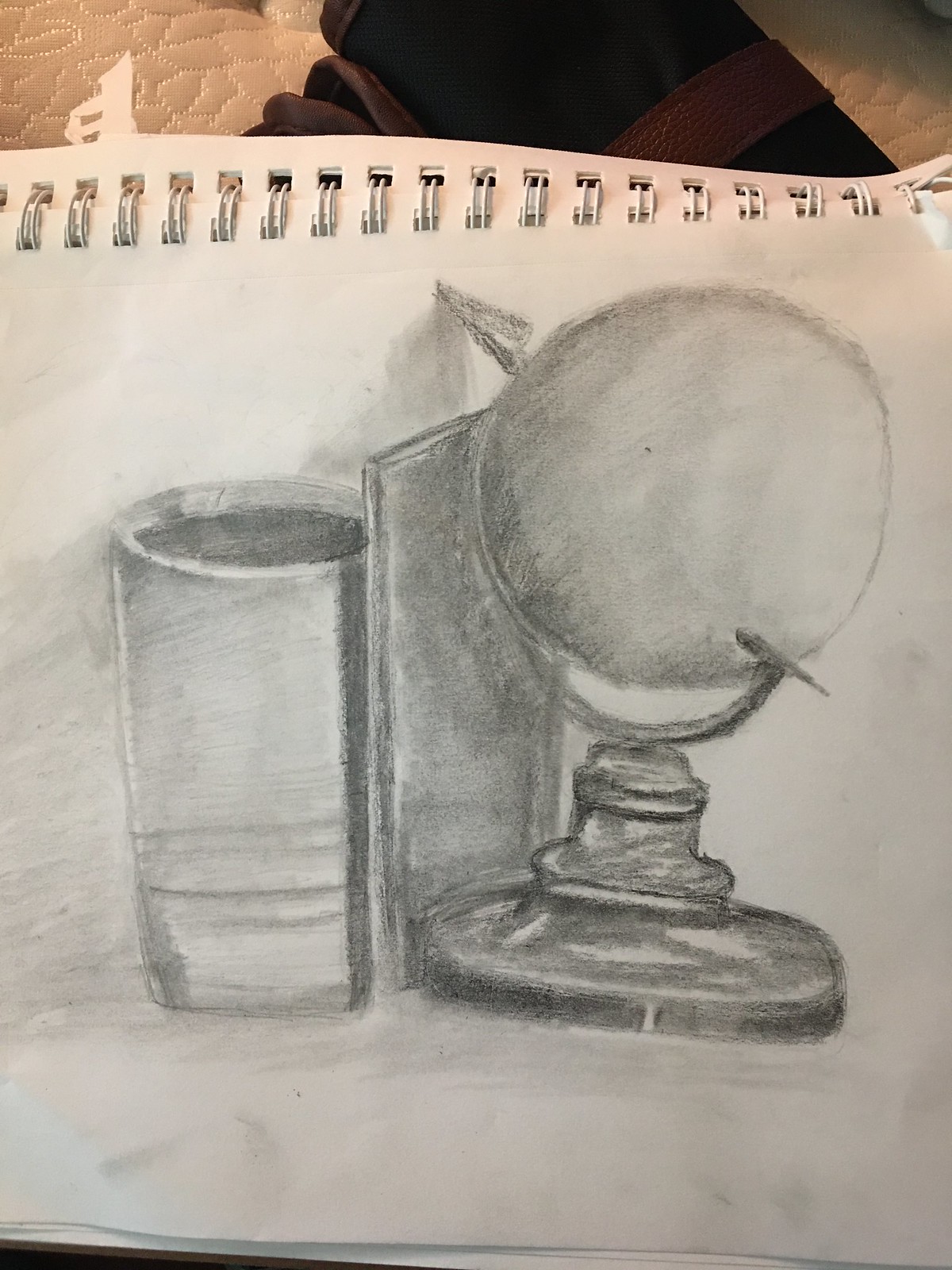This detailed illustration is drawn on the unlined pages of a notebook, with each sheet held together by a conspicuous white metal spiral binding. The artwork, created in pencil, depicts an intricate scene featuring a globe and an assortment of objects. Central to the drawing is a rounded base that gracefully narrows as it ascends, leading to a prominent arm that supports a globe at its midpoint. The globe itself is pierced by an arrow, adding a dynamic element to the composition. Adjacent to the globe stands a vertical book, and next to the book is a glass, which is notably darker on the inside than on the outside, adding a sense of depth and contrast. Above this central arrangement, the image captures a brown and black bag resting on a white mattress protector, providing a textured backdrop that contrasts with the central elements of the drawing.